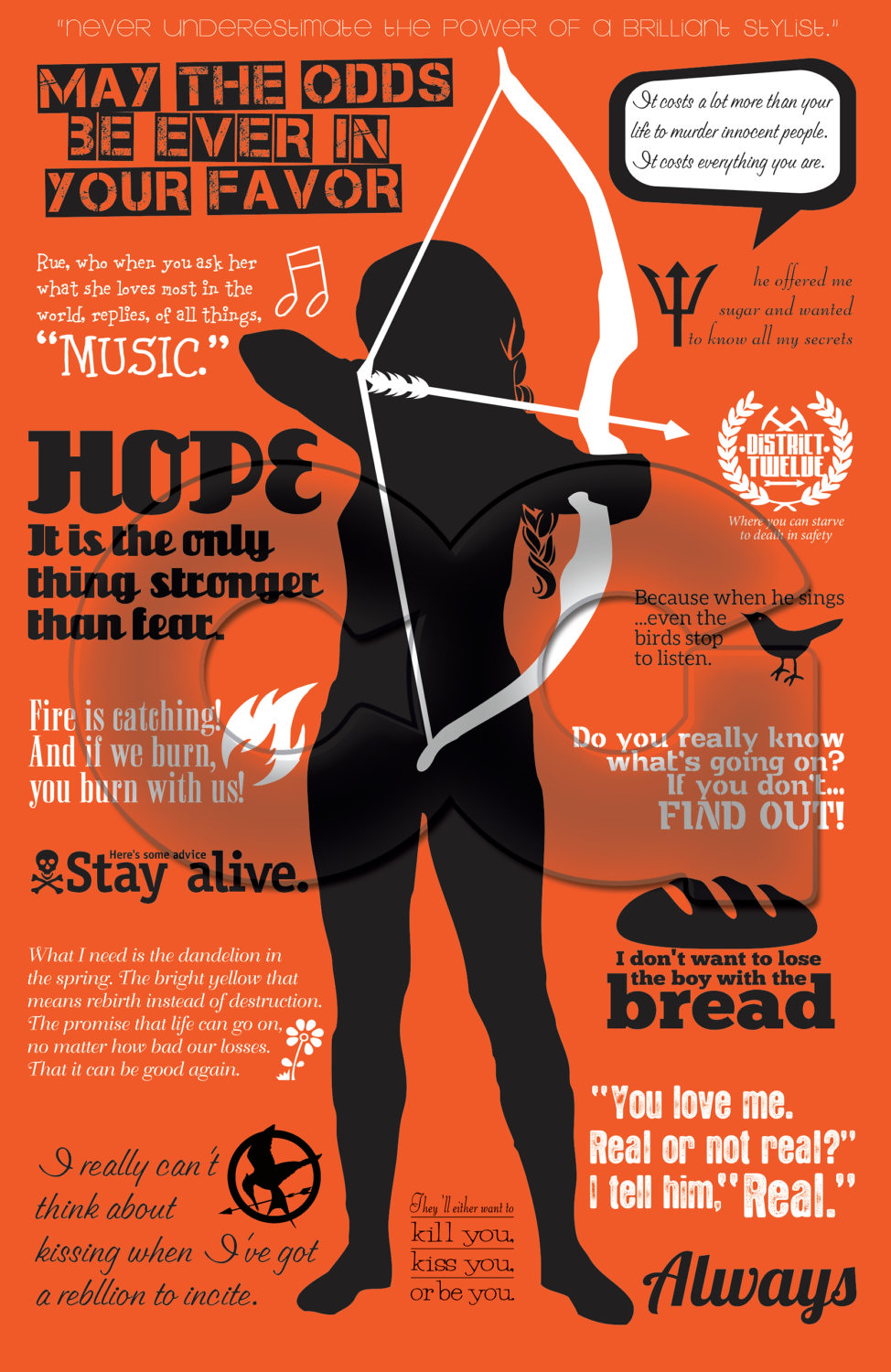The promotional flyer features an orange background with an eye-catching silhouette of a woman in black, holding a white bow and arrow, poised to release. Her ponytail is braided, and her details remain shadowed, emphasizing her form rather than her features. Surrounding her in various fonts and alternating black and white text, are a multitude of quotes and phrases. Notable quotes include "May the odds be ever in your favor," "Hope, it is the only thing stronger than fear," and "Here's some advice. Stay alive." Each quote is accompanied by corresponding icons, such as a white music note, a stylized flame, and a skull with crossed bones. Additionally, there's a faded overlay of the letters "C" and "Q" in the center. The flyer seems to promote an archery event, possibly focused on women, considering the emphasis on archery-related imagery and motivational quotes, although the exact purpose is not explicitly stated.